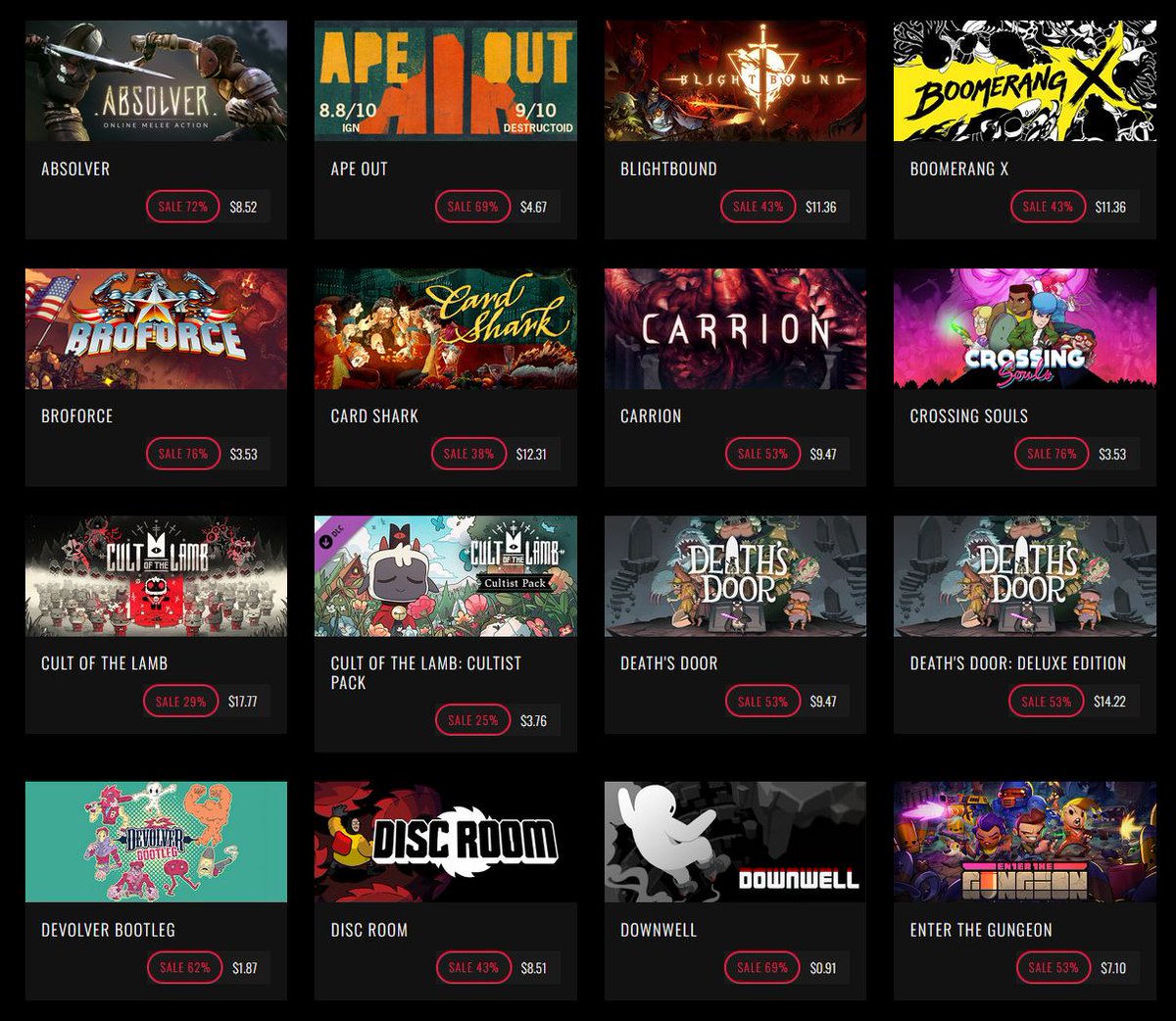The image showcases a digital game download platform with a black background featuring a grid of games, totaling 16 titles. The layout is organized in a left-to-right, top-to-bottom format. Each game is displayed with its cover art, name, price, and sometimes reviews or discount information. Here's a detailed breakdown of the games:

1. **Absolver**: The cover depicts two characters wearing what look like fencing masks, engaged in combat with swords. The game is on sale for $8.52, marked down by 72%.
   
2. **Ape Out**: The cover features an orange ape behind bars or in a cage. It’s highlighted with review scores, including an 8.8/10 from IGN and a 9/10 from Destructoid. Priced at $4.67.
   
3. **Blightbound**: The cover shows a sword intertwined with the title and depicts knights and dragons in the background. Available for $11.36.
   
4. **Boomerang X**: The cover is predominantly yellow with a large black X, accompanied by a black-and-white logo. It's priced at $11.36.
   
5. **Broforce**: Featuring an American flag and exaggerated soldiers, this game is available for $3.53.
   
6. **Card Shark**: A game with animated-style artwork on its cover.
   
7. **Carrion**: Available for $9.47.
   
8. **Crossing Souls**: Priced at $3.53.
   
9. **Cult of the Lamb**: Available for $17.77.
   
10. **Cult of the Lamb Cultist Pack**: Priced at $3.76.
   
11. **Death's Door**: Available for $9.47.
   
12. **Death's Door Deluxe Edition**: Priced at $14.22.
   
13. **Devolver Bootleg**: This game is on sale for $1.87.
   
14. **Disc Room**: The cover shows numerous saw-like discs, indicating a gameplay mechanic that likely involves dodging the discs. Priced at $8.51.
   
15. **Downwell**: The artwork features a ghost-like figure descending a well, rendered in black and white. This game is available for $0.91.
   
16. **Enter the Gungeon**: The cover art has a Japanese animation style with diminutive characters. Priced at $7.10.

Each game's cover art provides a glimpse into its theme and style, with prices varying across titles.